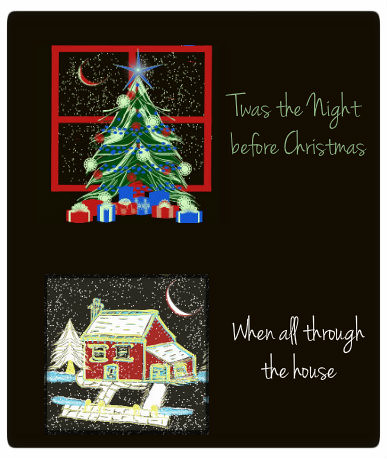The image is a digitally-created Christmas card artwork set against a black background. At the top left, it depicts a festive scene where a green Christmas tree adorned with a large blue star, blue garland, and white and red ornaments stands in front of a red-paned window. Through the window, a crescent moon and several yellow stars are visible, adding to the night-time ambiance. Beneath the tree, blue and red presents are neatly wrapped. The phrase "'Twas the night before Christmas" is prominently displayed in green text next to this scene.

On the bottom left, another image features a red house with a white and green roof set on a snowy street. A white tree stands outside to the left, framing the house. Above, a crescent moon shines brightly in the sky, surrounded by numerous stars. This scene is accompanied by the text "'Went all through the house," completing the festive narrative.